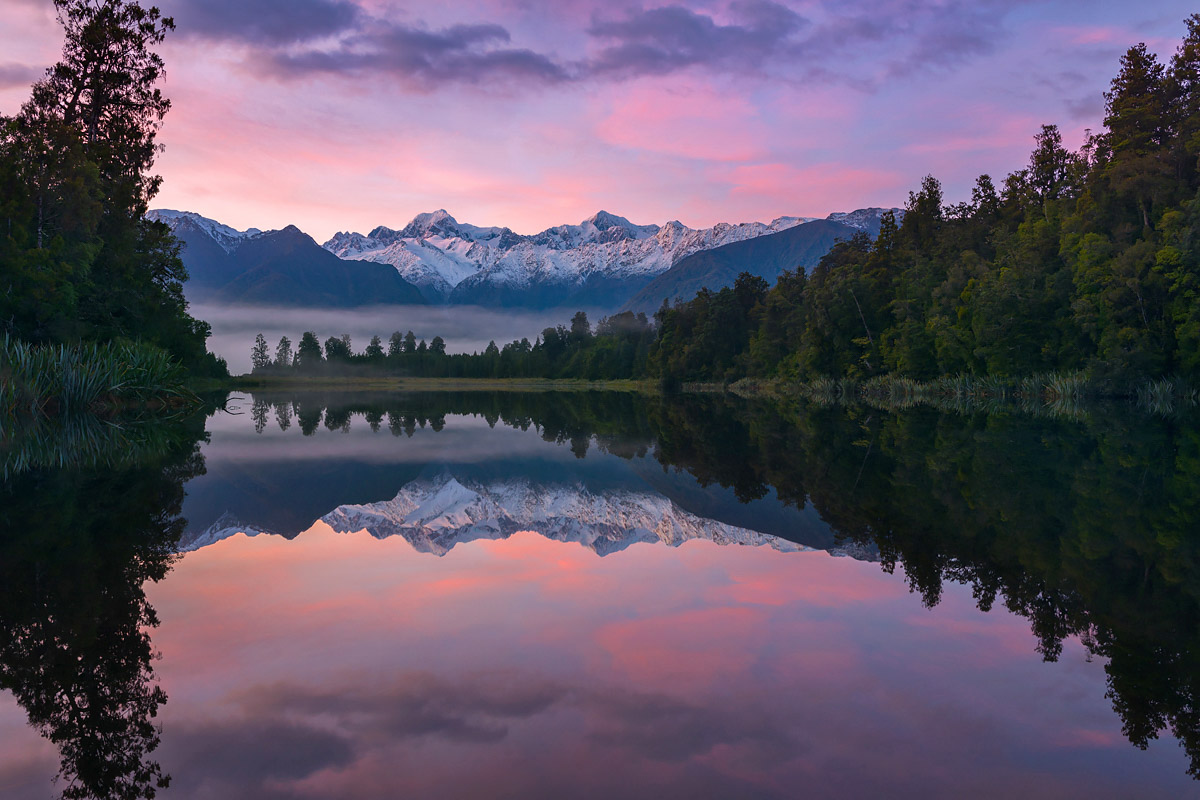This is a stunning wide-angle photograph capturing a serene lake set against a background of snow-capped mountains. The calm surface of the lake, occupying the bottom and middle parts of the image, beautifully reflects the surrounding scenery, including green pine trees and the sky. The trees, especially abundant and lush on the right side, gradually diminish in size and density as they extend towards the left and to the far distance. The landscape features a ridge that stretches across the entire backdrop, showcasing rugged mountain edges dusted with snow. Above these mountains, the sky displays a harmonious blend of blue hues interspersed with pink and purple clouds, illuminated by the soft glow of the setting sun, which is partially visible on the top left. A layer of gray and white fog rests beneath the mountains, adding a mystical touch to the scene's overall composition. The scene is bathed in the muted, tranquil light of dusk, with the vibrant sunset colors creating a striking contrast against the darker tones of the trees and reflecting on the water's glossy surface.